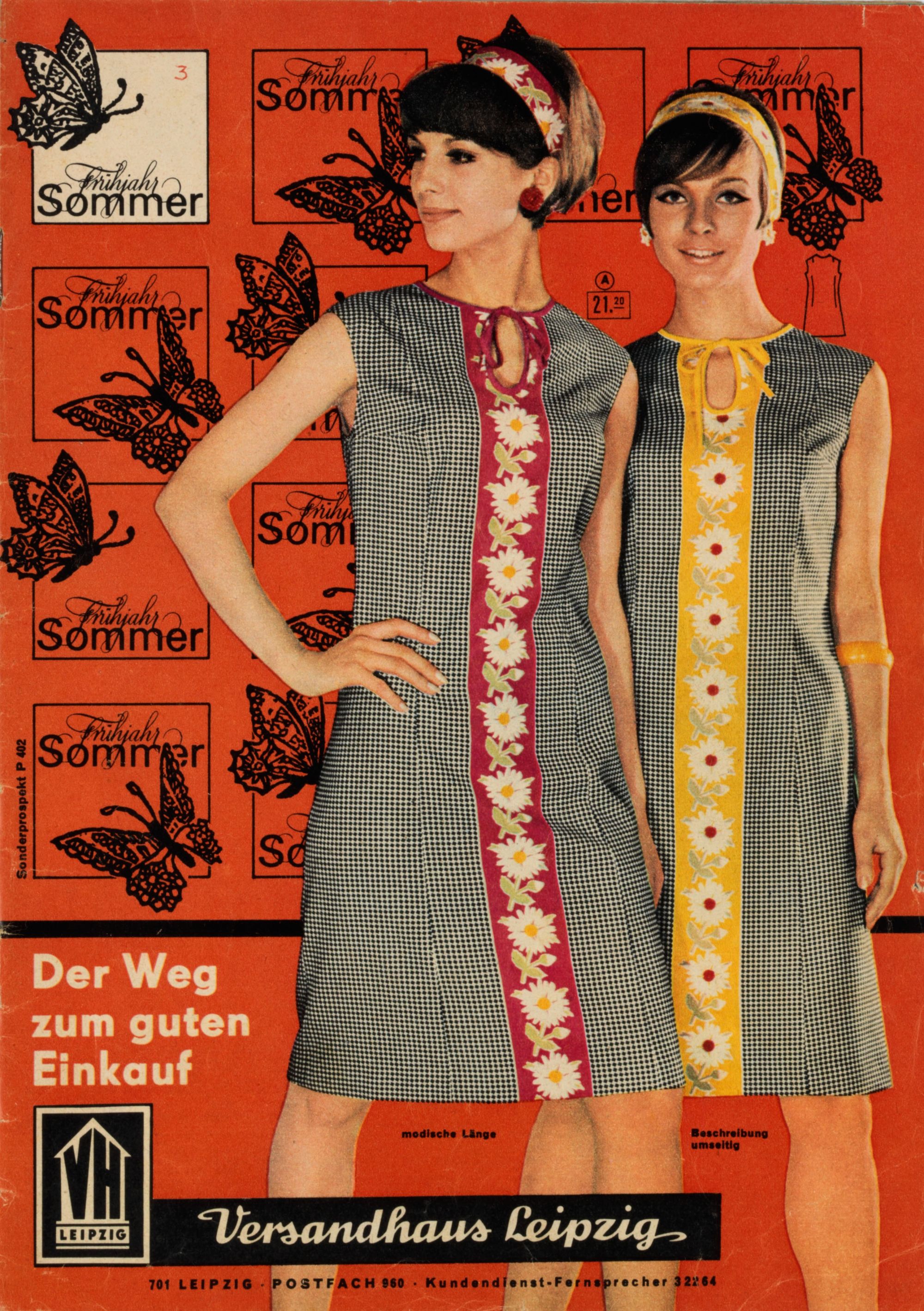This image is a vintage fashion advertisement from what appears to be the 1960s, featuring two young women modeling floral dresses. The background is a bold reddish-orange with black butterfly illustrations, lending an artistic and slightly nostalgic feel. 

The woman in the center has short dark brown hair adorned with a red floral headband. She is wearing a sleeveless black-and-white checkered dress that reaches her knees. This dress has a striking red floral stripe running vertically down its center, complete with detailed white flowers, green stems, and yellow pollen. Her right arm is placed confidently on her hip, and her head is slightly tilted to the right.

Standing just behind her to the right is another woman with similar short dark brown hair, decorated with a yellow floral headband. Her dress is identical in style and pattern, but features a yellow floral stripe instead of red. She also sports a gold bangle around her left elbow. Both women have sleeveless dresses that tie around the neck with matching colored ties—red for the woman on the left and yellow for the woman on the right.

The text on the poster is in German, with phrases like "Schingham Summer, Der Weg zum guten Einkauf" prominently displayed. Additional text includes locations such as "Versailles, Haas, Leipzig," and other details like "Lesbink, Postfotch, 860, Huden, Neist, Werner Preacher, 32264." All of this is framed by a black border at the bottom of the advertisement.